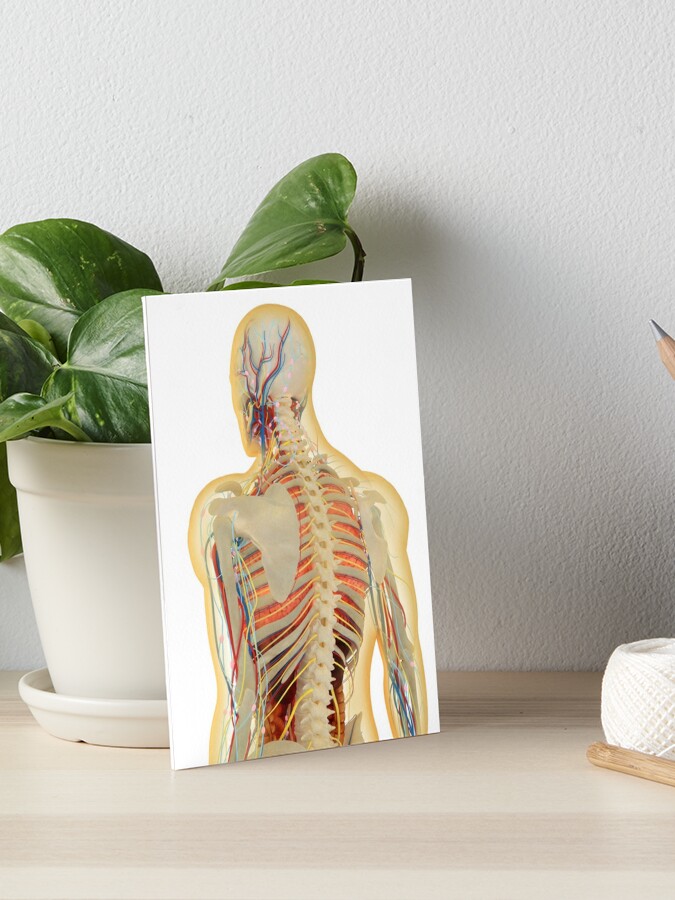The image features a meticulously staged scene resembling a stock photo used for display purposes. It showcases a neutral, minimalist environment with a light wood shelf and bright white walls, creating a clean, uncluttered backdrop. A small, common indoor house plant in a white pot sits on the shelf, with its green leaves providing a touch of nature to the setting. 

Peeking into the corner of the photo is a pencil holder filled with visible pencils, adding a subtle, practical detail to the composition. Another notable element is a spool of white thread, contributing to the scene's simplicity and brightness.

Leaning against the plant is a detailed picture of a human skeleton, with its back oriented towards the camera. The skeleton image is transparent, allowing viewers to see an intricate overlay of muscles, nerves, veins, and internal organs. Red and blue lines illustrate the veins and arteries extending from the arms, while yellow lines trace the spinal cord and nerves throughout the body, culminating in a complex web of blue, red, and yellow veins and nerves within the head. This photo seems digitally inserted to serve as a product display image, possibly for an educational or medical website.